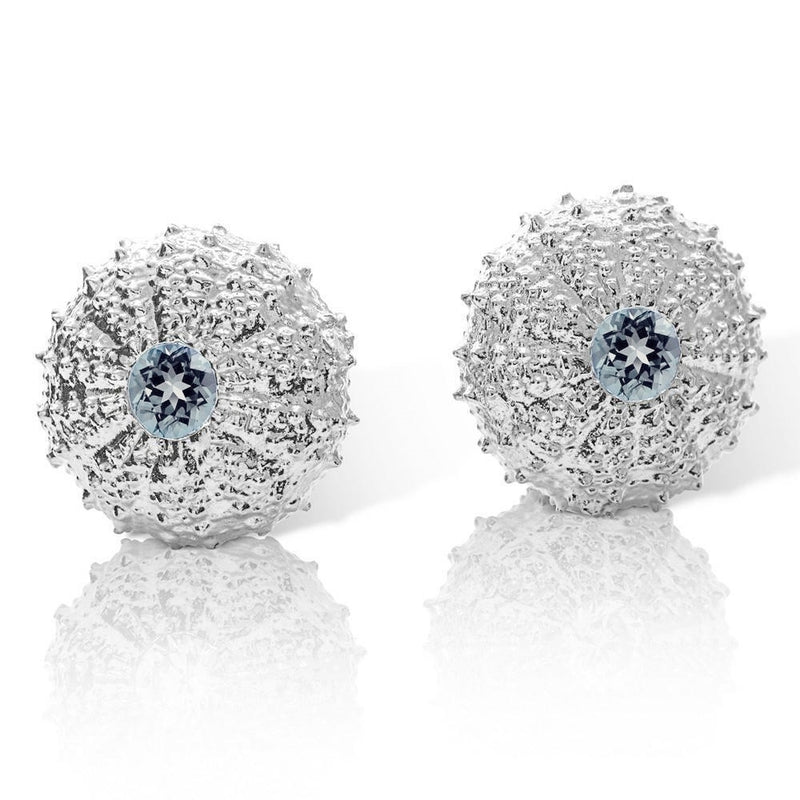The image features two spherical objects that closely resemble spiky, chrome chestnuts or sea urchins, potentially serving as earrings or cufflinks. These objects exhibit a detailed design, with cylindrical patterns formed by silver-like metal or stone. At their center, a starburst or floral shape radiates with dark navy, white, and light blue hues, creating a striking contrast. The objects are three-dimensional, rounded, and completely solid, devoid of any holes. The intricate surface resembles a spiderweb or beach ball pattern with spikes, adding to their ornate appearance. Set against a stark white background, the items have a mirrored reflection below them, further emphasizing their glossy, reflective quality and enhancing the overall visual impact.